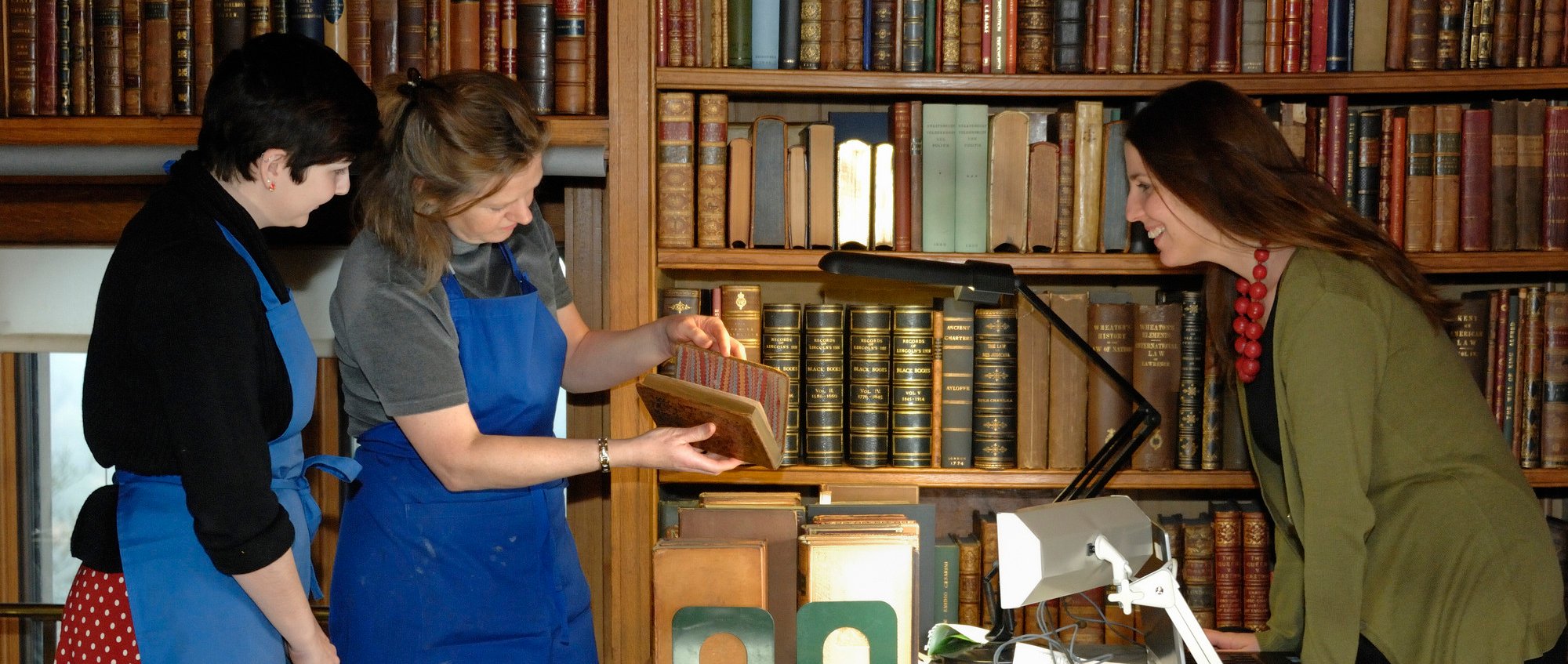In this image, three women are gathered in a library, standing next to a wooden desk laden with typical office paraphernalia such as bookends and two desk lamps—one black and one white, both illuminating the scene. Behind them, a backdrop of wooden bookshelves filled to the brim with books stretches across the frame. The woman on the far right is dressed in a light green khaki sweater over a black blouse, accessorized with a red beaded necklace. She has long brown hair cascading down her back and appears to be leaning forward against the desk, smiling at a book. On the left, two women in blue aprons stand side by side. The woman in the center is clad in a gray t-shirt beneath her apron and is holding a partially opened book, to which all three women direct their gazes. The other woman on the left dons a black long-sleeved blouse under her apron with a red and white dress peeking through. She sports short dark hair and, like her companions, is smiling at the book. The scene exudes a warm, collaborative atmosphere typical of a vibrant, bustling library.